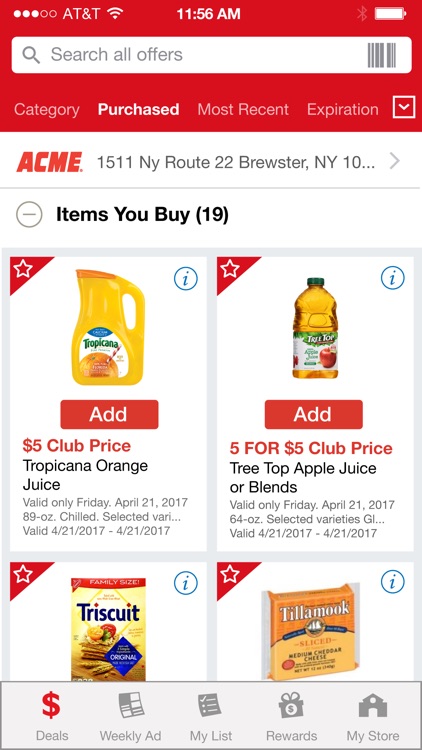The image depicts an advertisement for Acme displayed on a smartphone screen. The background of the ad is predominantly red. It is 11:56 AM, as indicated by the phone's status bar, which also shows a full battery, AT&T as the service provider, and three out of five signal bars filled. At the top of the screen, there is a search bar labeled "Search all offers" and a clickable skew box.

The screen appears to show a categorized list, with options like "Category," "Purchased," "Most Recent," and "Expiration." The "Purchased" category is currently selected, as it is highlighted in bright white compared to the other options, which are in a fainter white shade.

Below the categorization options, the ad specifies the store's location: "Acme, 1511 NY Route 22, Brewster, New York," followed by an ellipsis. There's an icon resembling a circle with a minus sign, indicating a list of items the user has bought, which totals 19 items. 

The visible items include:

1. Tropical Orange Juice
2. Treetop Apple Juice for Blends
3. Triscuit Crackers
4. Tillamook Cheese

Each item is displayed with a picture and has an "Add" button next to it for adding the item to a shopping cart.

At the bottom of the screen, there are menu options labeled "Deals," "Weekly Ad," "My List," "Rewards," and "My Store," suggesting various functionalities that the user can explore on the app.